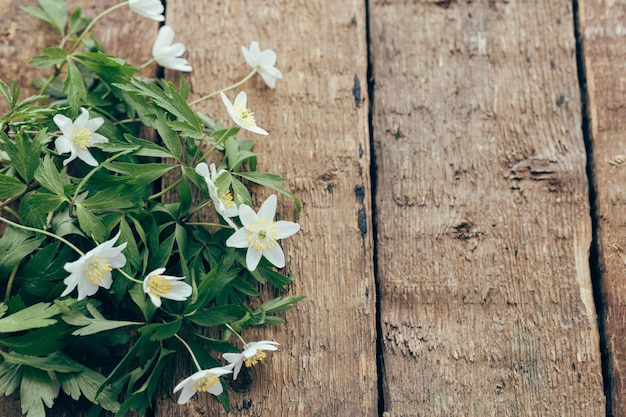A photograph capturing a rustic scene where the right-hand side features a rough, unfinished wooden plank surface. The texture of the wood is evident, suggesting it could be from a picnic table, board, or fence, characterized by its unvarnished, unsanded, and natural state. On the left-hand side, a vibrant bouquet of flowers rests atop the wooden surface. These flowers, resembling daisies, each boast six white petals encircling a central section filled with small, yellow, pollen-coated stamens and a slightly greenish core. The bouquet displays at least eleven visible blooms, interspersed with abundant green leaves, adding a touch of natural elegance to the contrasting raw wood.